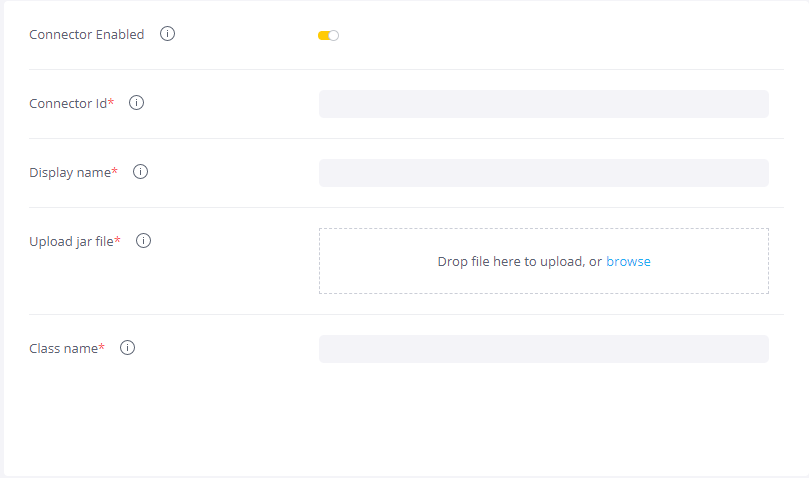**Caption:**

The image displays an interface for uploading a file or configuring settings. Located in the upper left-hand corner, there is a toggle switch labeled "Connector Enabled," which is turned on. Below this, the interface presents a set of fields against a white background with grey entry bars, each accompanied by red asterisks indicating they are required. The fields include "Connector ID," "Display Name," "Upload Jar File," and "Class Name."

- **Connector ID**: Currently blank.
- **Display Name**: Currently blank.
- **Upload Jar File**: An area that reads "Drop file here to upload or browse," with a "Browse" hyperlink in blue text, indicating that no jar file has been uploaded.
- **Class Name**: Also currently blank.

Each field includes an information icon (an "i" inside a circle), suggesting that additional information is available for users who need further explanation.